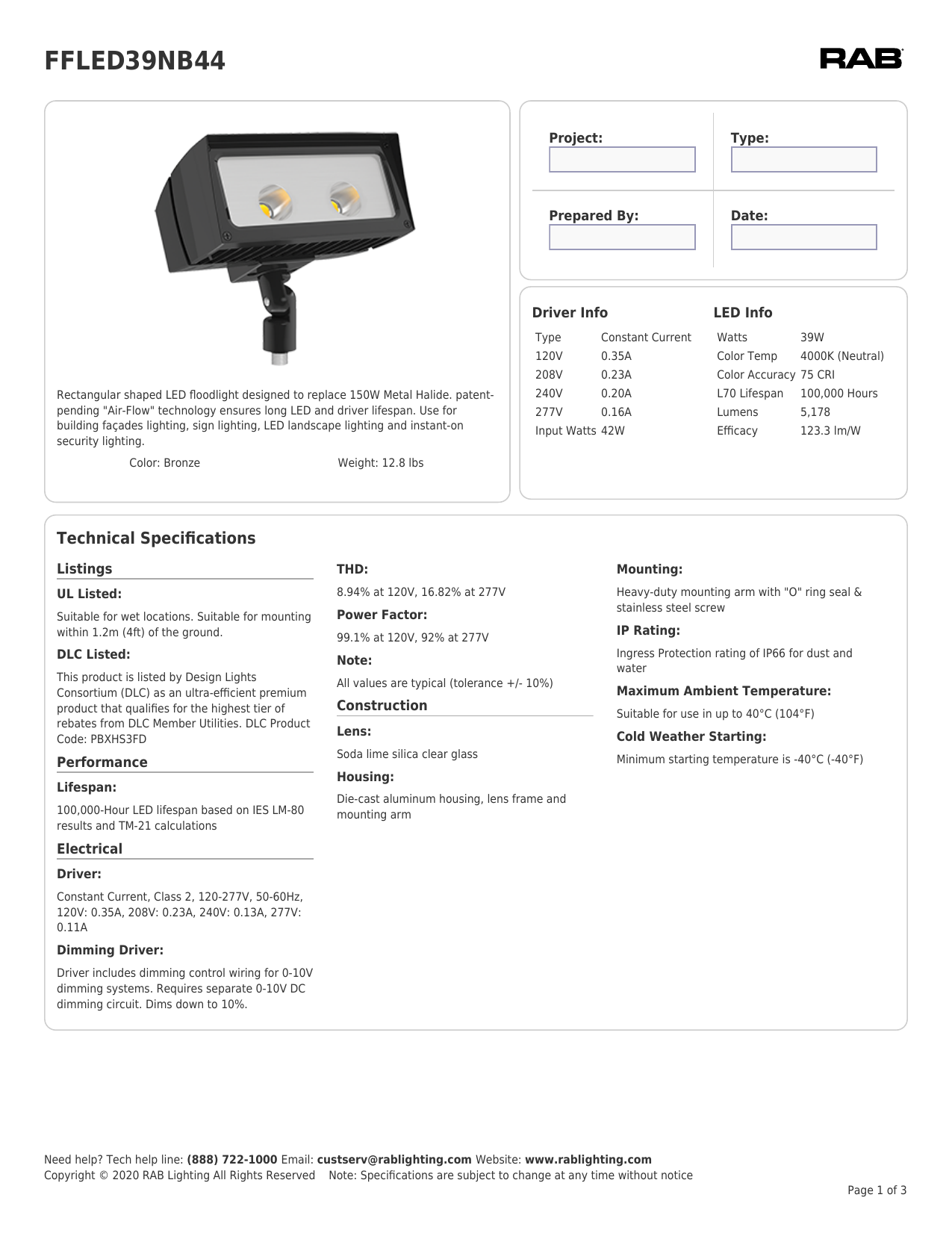This image appears to be a detailed technical data sheet, likely a screenshot from a tablet or laptop, showcasing the specifications of the FFLED39NB44 LED floodlight, produced by RAB Lighting.

The floodlight itself is designed with a bronze-colored, rectangular frame and contains two internal light sources. It is intended to replace a 150W metal halide light and features a patented airflow technology that ensures a long lifespan for both the LED and the driver. This versatile light is suitable for various applications such as building facades, sign lighting, landscape illumination, and instant-on security lighting. The product details are comprehensively outlined, including its weight of 12.8 pounds.

Key technical specifications are provided as follows:
- **LED Info**: It operates at 39 watts with a color temperature of 4000K (neutral white) and a color accuracy (CRI) of 75. The L70 lifespan is rated at 100,000 hours, delivering 5178 lumens with an efficacy of 123.3 lumens per watt.
- **Driver Info**: It uses a constant current driver compatible with voltages from 120V to 277V. Power consumption details are listed for various voltages (e.g., 42 watts at 120V). The driver also supports dimming from 0-10V systems, down to 10%, with specific harmonic distortion and power factor values.

The product is UL listed for wet locations and suitable for mounting within 1.2 meters (4 feet) from the ground. It is also DLC listed, qualifying for the highest tier of rebates from the Design Lights Consortium member utilities. The DLC product code is PBXHS3FD.

Construction details include a soda lime silica clear glass lens, die-cast aluminum housing, and a robust mounting arm with an O-ring seal and stainless steel screws. The floodlight is rated IP66 for dust and water ingress protection, operates in ambient temperatures up to 40°C (104°F), and can start in cold conditions down to -40°C (-40°F).

For technical support, the document provides a Tech Line (888-722-1000) and an email address (CUSTSERV@rablighting.com). More information can be found on the RAB Lighting website (www.rablighting.com). This document is copyrighted in 2020 by RAB Lighting, and specifications may change without notice. This image is labeled as page 1 of 3.